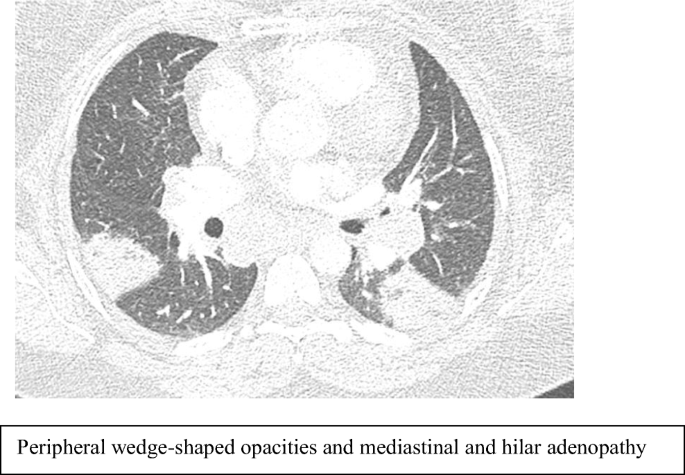This image appears to be a scientific illustration, likely a pencil drawing that has been photocopied in black and white. The drawing is grainy and low-resolution, resembling a cross-sectional x-ray of a human torso. Central to the image are two lung-shaped figures, illustrated in varying shades of gray, with darker tones on either side. These lung-like shapes are surrounded by an oval white band, which contrasts the whitish background and various white circles and splotches interspersed between the two darker sections. The overall composition is light gray and slightly fuzzy, indicating it might have been produced with limited resolution. At the bottom of the image, in black ink, are the medical terms "peripheral wedge-shaped opacities" and "mediastinal and hilar adenopathy," suggesting that the illustration is highlighting specific pathological features in the organ system depicted.